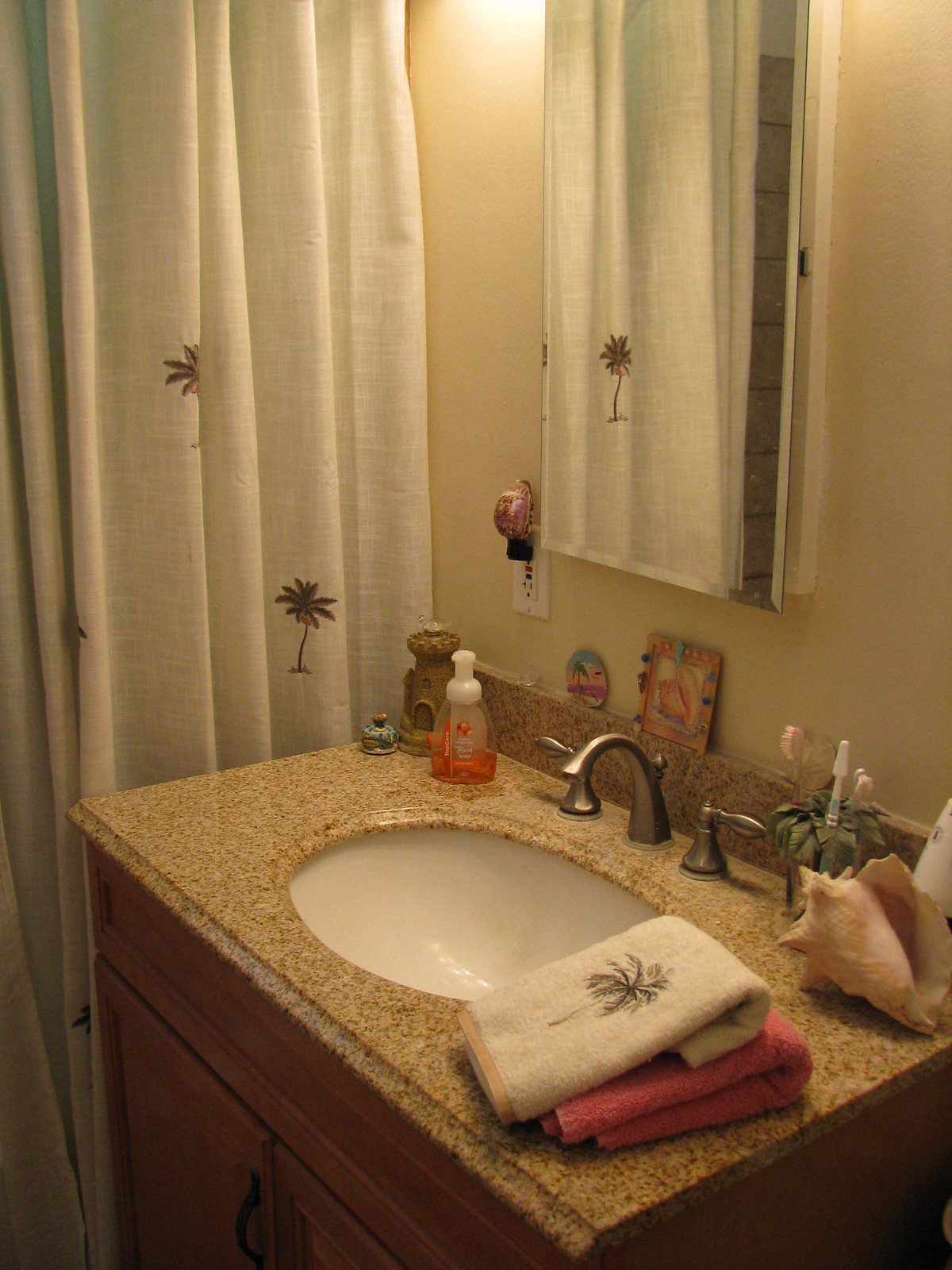The photograph features a well-organized bathroom sink setup. At the forefront, there's a brown wooden cabinet supporting a countertop with brown speckled patterns, possibly made of porcelain or similar material. It holds a glossy white basin. The chrome faucet has distinct left and right levers for hot and cold water.

On the countertop, a couple of neatly folded face towels can be seen. The bottom towel is peach-colored, while the top one is white, adorned with a palm tree design in the center and a gold band at its end. Behind these towels, a large decorative seashell rests.

To the left of the towels, there is a toothbrush holder resembling a cup with decorative leaves, from which four toothbrushes protrude. Directly left of the faucet, a white pump dispenser contains orange hand soap.

Adjacent to these items on the left are more decorative pieces, including a small lighthouse figurine and a blue, round object. The backsplash of the sink area features a speckled pattern of brown and tan. It supports a few small square etchings with vibrant, Aztec-like designs, leaning against the light tan wall.

Also on the backsplash, a circular decorative piece depicts a beach scene with a palm tree, blue sky, and sandy shore. Next to this artwork, there's a white electrical receptacle with red and black safety buttons, likely to prevent water-related incidents. A nightlight with a shell design is plugged into this receptacle.

Above the sink stands a medicine cabinet with a slightly open horizontal glass door, revealing the magnetic latch in the middle. To the far left, a white shower curtain adorned with palm tree motifs is partially visible, adding to the tropical ambiance of the bathroom.